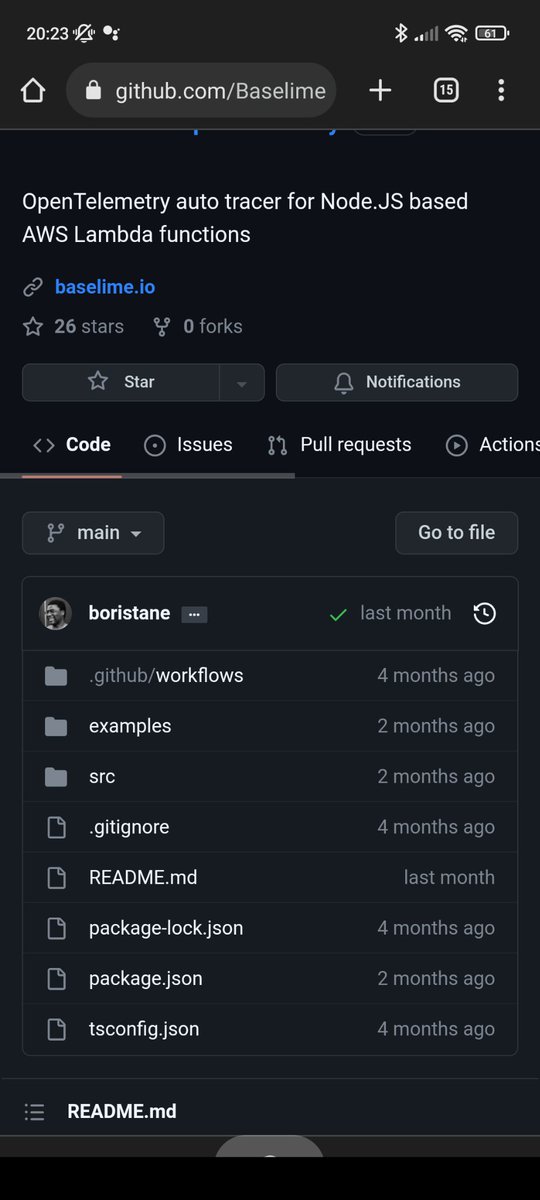This is a detailed screenshot of a GitHub repository page for "OpenTelemetry Autotracer for Node.js-Based AWS Lambda Functions." 

In the mobile view:
- The status bar is black, displaying the time "20:23" in military format on the top left and a battery icon indicating 61% charge on the top right.
- The web address bar reads "github.com/baseline," with a plus sign and an icon showing that 15 tabs are currently open.
- The webpage itself features a black background.

Key details on the page include:
- A prominent display name in white text: "OpenTelemetry Autotracer for Node.js-Based AWS Lambda Functions."
- A chain icon followed by "baseline.io" in blue, indicating a link.
- A star icon indicating the repository has 26 stars and zero forks.
- Below the star icon are two buttons: a "Star" button to the left and a "Notifications" button to the right.
- The content is organized into four columns with the "Code" column selected on the left.

Highlighting the "Code" column:
- Below the main navigational menu, the first entry shows the username "orstein" with a timestamp labeled "last month" and a checkmark next to it.